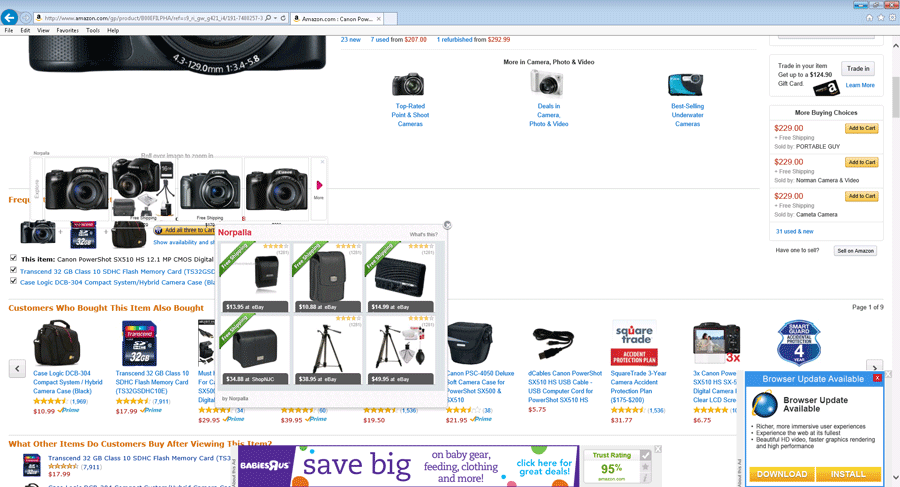Page Caption: 

This image depicts a web browser window open to a single active tab, showcasing an Amazon.com product listing. The URL at the top reads "www.amazon.com," indicating it is an Amazon webpage. Below the URL bar, the browser's menu options—File, Edit, View, Favorites, Tools, and Help—are visible.

The main content of the page features various camera-related items. At the top section of the page, the Amazon logo and URL are clearly visible, along with an incomplete image of a camera, suggesting the page allows for vertical scrolling. Various smaller icons of additional camera models and accessories, such as memory cards, bags, and cables, are scattered throughout the page. A specific section titled "Customers who bought this item also bought" showcases similar and complementary products.

To the right of the screen, there are purchasing options like pricing details and an "Add to Cart" button, with more choices listed at $229. The bottom right corner displays a browser update notification, advising to "Download and Install," which appears to be a system prompt rather than a website feature. At the very bottom, an advertisement for Babies R Us is displayed.

Based on the content and layout, this page appears to be listing details for a Canon camera on Amazon.com.